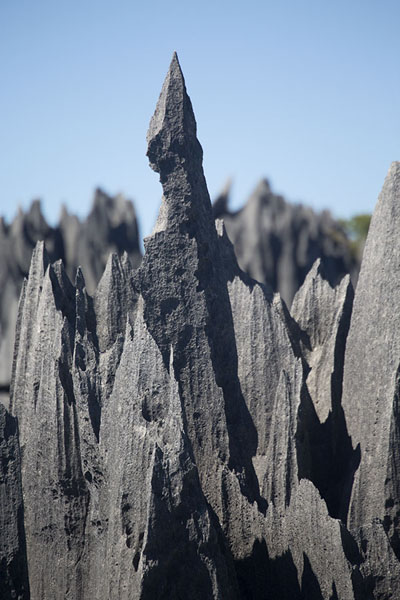This close-up photograph captures a dramatic rock formation, showcasing a collection of jagged, dark gray to black rocks that dominate the frame. The subject is framed from ground level, emphasizing the sharp, spiky contours that rise vertically. The rock in the center, appearing almost black with the sun reflecting off parts of it, pierces dramatically into the top middle of the image, resembling a turret. This central rock is the tallest and most pronounced, with other spiky rocks branching out towards the right. Behind this focal point, slightly out of focus, lies more of the rugged formation, creating a layered, almost spear-like arrangement. The backdrop of the scene is a clear, light to medium blue sky occupying the upper quarter of the image, accentuating the stark, natural beauty of the rocks with no clouds in sight. The texture of the rocks looks extremely sharp and rough, appearing as if they could cut through anything that touches them. The whole composition underlines the rugged and majestic nature of this natural formation against a serene, sunny sky.